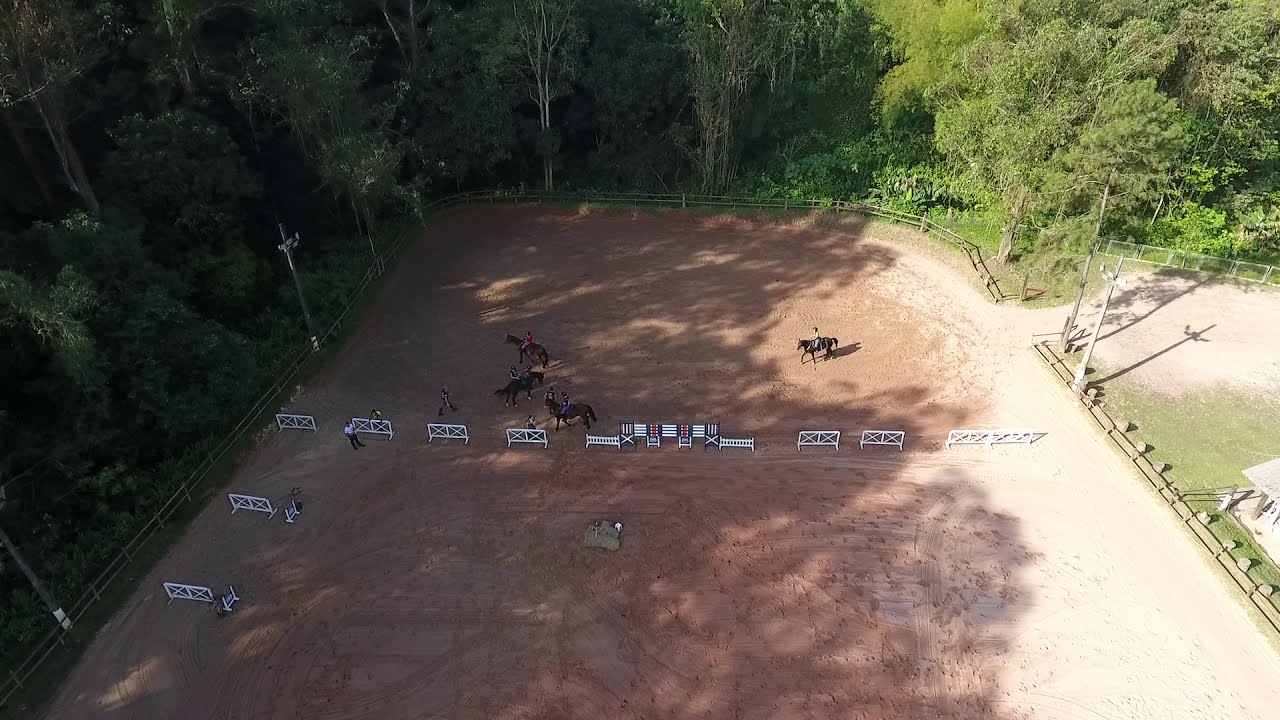The image depicts a large, outdoor equestrian arena set up for horse jumping and dressage events. The ground is entirely covered in dirt, and the arena features approximately ten white barriers arranged for the horses to jump over. Most of these barriers are uniform, rectangular with crosses in the middle, while some central taller barriers have four poles, with white exteriors and sections in the middle colored red and gray.

Several horses, primarily brown and black, are visible near the first line of barriers, accompanied by a few people, including one in a white shirt and black pants, who appear to be guiding and possibly training them. The arena is encircled by thick, tall green trees, with sunlight illuminating the foliage on the top right side of the image and casting shadows on the top left. There is a brown wooden fencing that outlines the arena, with an entrance on the far right leading to a small dirt opening and a parking lot area with patches of green grass beyond.

Overall, the image offers a detailed overhead view of an active horse.